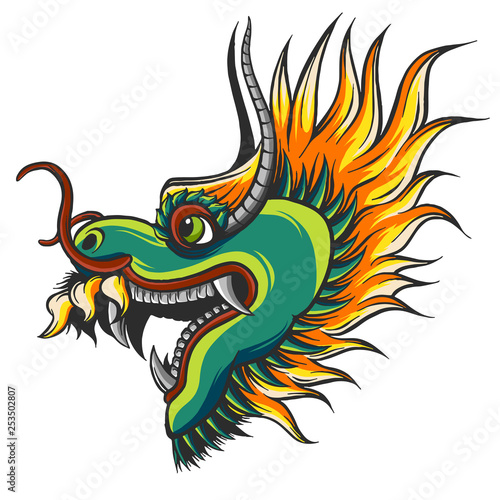The image showcases a detailed, animated head of a dragon oriented to the left side. The dragon's face features a rich palette of blue, bluish-green, and green hues. Its formidable mouth is filled with an array of sharp teeth, including elongated fangs on both the top and bottom rows. A notable feature is the dragon's eye, which is a striking green. Gray horns protrude from above the eye and additional horns are seen coming off its nostrils. In contrast to the cool tones of its face, the dragon's mane bursts into vibrant flames of orange and yellow that extend behind its head. The snout includes red squiggly accents and hints of fire emit from its mouth, adding a dynamic fiery effect. The dragon also has tufts of yellow and orange fur near the front of its mouth over the gray fangs. The entire scene is set against a stark white background, with no additional text or setting details apart from some descriptive writing and an Adobe stock number in the corner.